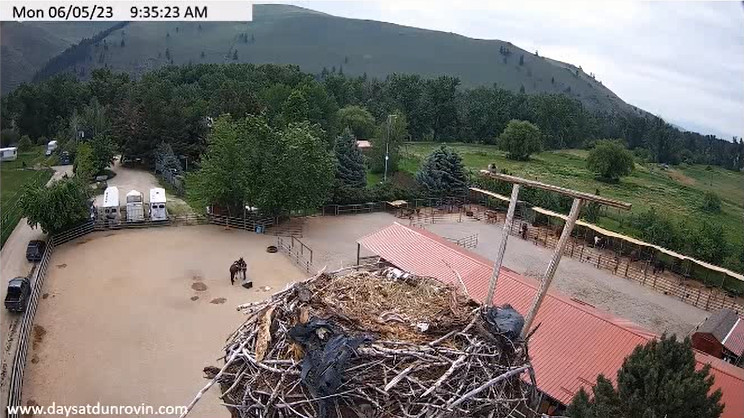Captured from a unique aerial view, this webcam image showcases a carefully constructed nest composed of twigs and branches, resting serenely with no occupant. The nest is accented with scattered pieces of plastic and a few strands of grass, hinting at an avian architect's resourcefulness. To the right of the nest, a small perch is evident, seemingly designed for a bird to rest or scout from. The backdrop reveals a charming ranch scene, complete with horse trailers, a corral, and a dedicated horse riding area. Shaded horse barns provide shelter, all framed by a picturesque mountain range, hillside, and scattered trees in the distance. In the upper left corner, the screen displays a typical webcam description, indicating the date as Monday, 06/05/23 and the current time as 9:35:23 a.m. The bottom left corner bears the logo and website www.daysatdonerobin.com, signifying the source of this serene pastoral snapshot.